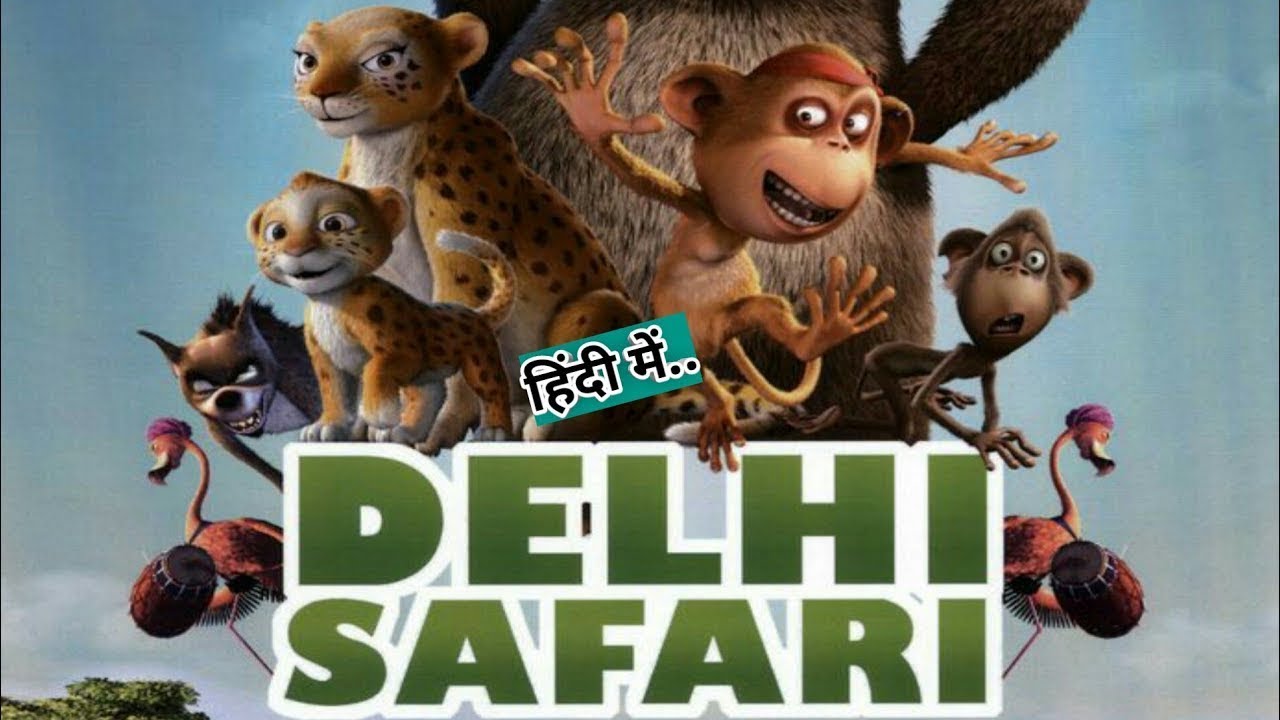The movie poster for the animated film "Delhi Safari" showcases a vibrant collection of illustrated animal characters against a vivid blue background with a green tree in the bottom left corner. Prominently featured at the bottom in large green letters with a white outline is the title "Delhi Safari," and above it, text in Hindi nestled on a green background. The lively ensemble includes two pink flamingos on either side, each adorned with hats and playing pink drums with red sides. Among the animals are a tan and black hyena with a white chest and around his mouth, a mother and baby cheetah with tan fur and black spots, and a pair of monkeys—one brown with a white belly and another with tan coloring around its face and belly. Dominating the rear of the group is a large bear-like figure with only its brown furry belly and hands on its hips visible, as its face is cut off by the poster's top edge.